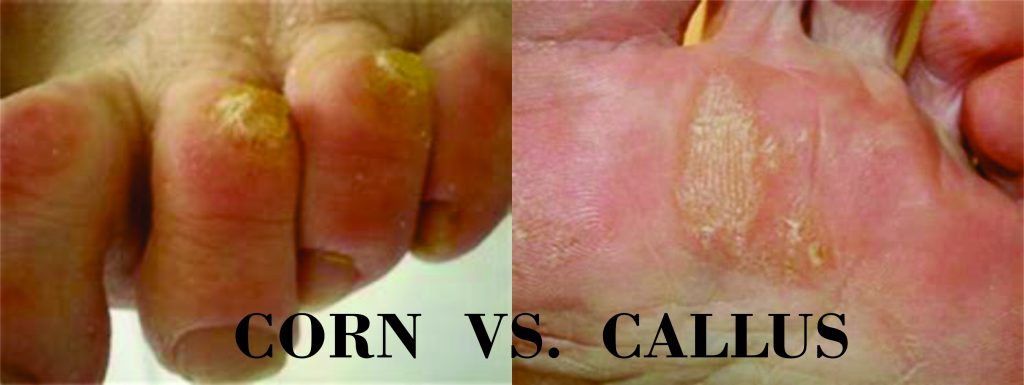The image is a landscape-oriented graphic divided into two halves, each illustrating different foot conditions. On the left, there is a close-up of four reddish, light-skinned toes, with prominent yellow corns appearing as postural masses on the knuckles of the middle toes. On the right, the image shows the bottom of a similarly reddened foot, featuring scaly skin and a cracked, yellowish-white callus in the center. At the bottom of the image, in all caps black text, the caption "CORN VS. CALLUS" stretches across both pictures, clearly explaining the visual comparison between corns and calluses, emphasizing the medical issues affecting the feet.